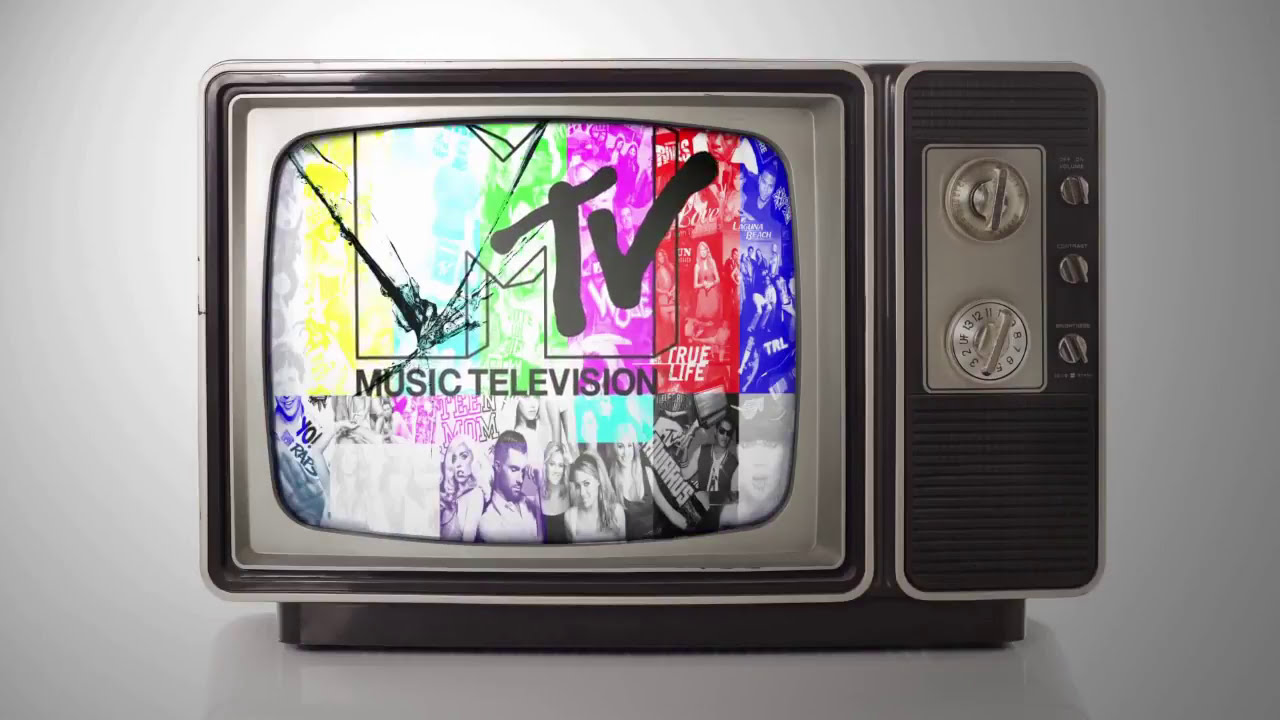The image showcases a meticulously rendered 3D depiction of a vintage CRT television, reminiscent of models from the late 1960s to the 1970s. The TV has a rectangular shape, with its body predominantly matte black, adorned with a contrasting silver border. The right side of the TV features two prominent silver knobs, accompanied by three smaller knobs, each reflecting a shiny surface against the duller black backdrop. The bottom knob has visible numbers that reach up to 13. The screen captures a colorful montage featuring the iconic MTV logo with the text "Music Television" beneath it. Various vibrant hues, including yellow, turquoise, purple, red, and blue, are prominently displayed as vertical sections superimposed with graphics that resemble bands and performers. The gray-scale background of the image transitions from light gray on the left and top to darker gray shades towards the bottom and right, framing the central focal point—the nostalgic television set.